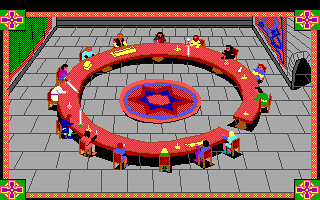This screenshot from the early 90s 2D video game "Conquest of Camelot" depicts a vibrant scene set inside a castle's chamber. Central to the image is a round table surrounded by figures seated in ornate chairs, likely representing the legendary Knights of the Round Table. The table's centerpiece is a striking orange mat adorned with a prominent blue six-pointed star, outlined in red, adding a mystical element to the composition. The floor is composed of meticulously arranged gray tiles, contributing to the medieval ambiance of the room. Adding further authenticity, colorful banners hang proudly from the stone walls, enhancing the regal atmosphere of this iconic Arthurian setting.